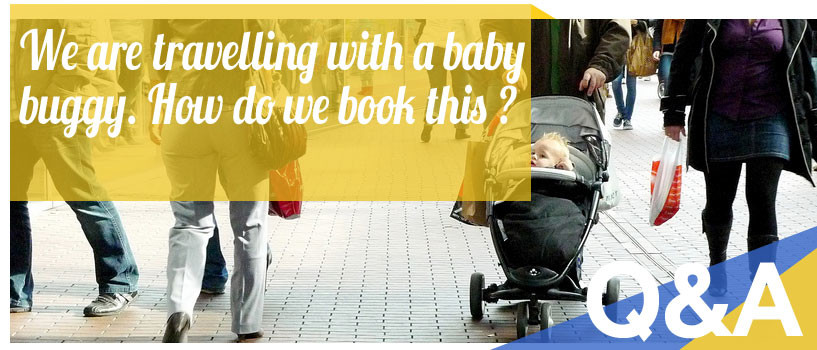The image depicts a busy outdoor scene with people walking on a gray brick sidewalk, suggesting a chilly day as they are wearing jackets. Dominating the center of the scene is a man pushing a stroller containing a blonde baby, who appears to be about eight months old. Standing next to the stroller is a woman carrying a distinctive red and white bag. The background is lively and crowded, possibly in a public place such as an airport or a mall.

Superimposed on the image is a light yellow area stretching from the left towards the right. In white font, it reads, "We are traveling with a baby buggy. How do we book this?" Additionally, the bottom right corner features an overlay with blue and yellow stripes, containing white letters in a Q&A format, including the text "Q," "& A," and "Q and A." This is likely a marketing piece designed to address travel inquiries involving baby carriages.